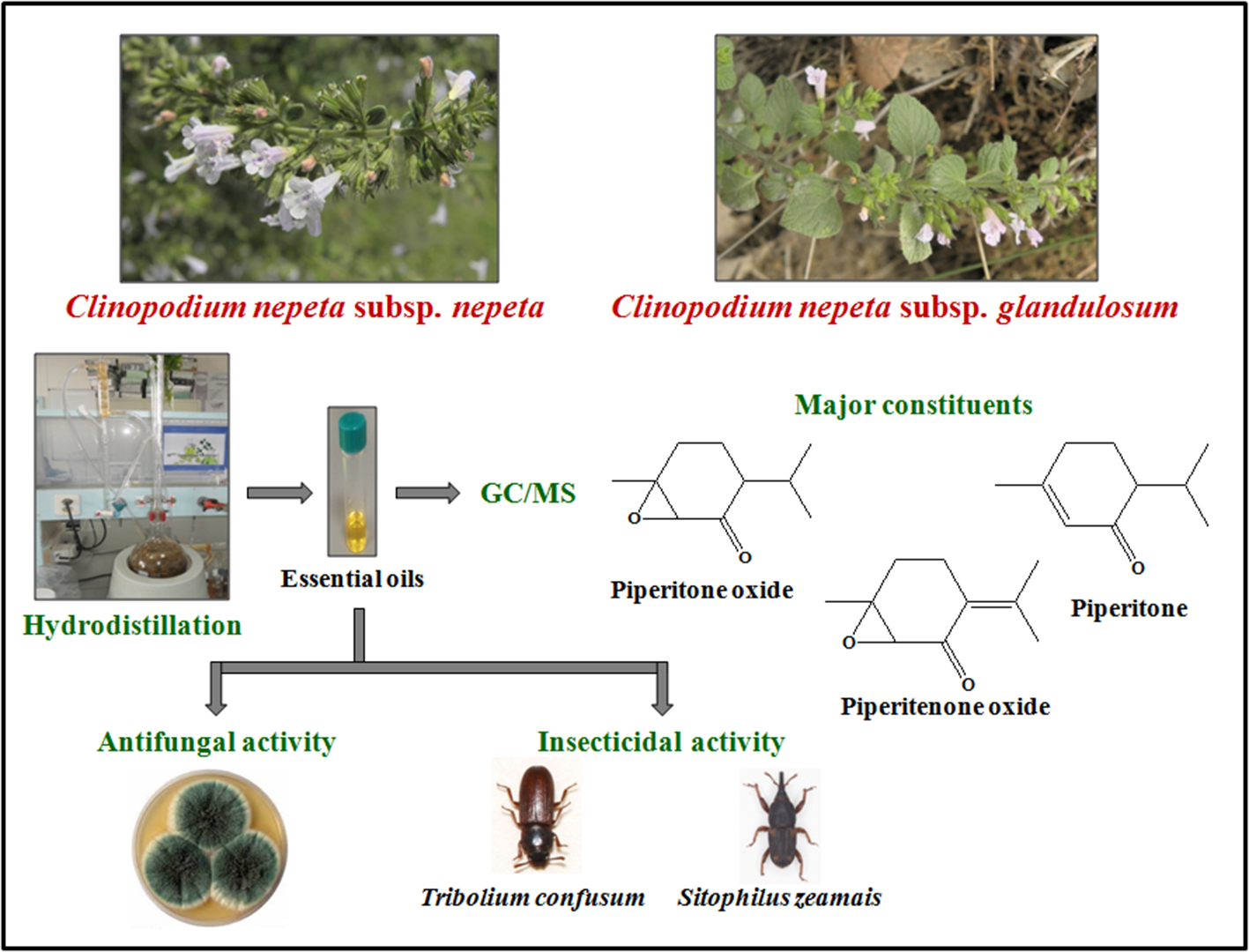The image, likely from a science lecture, prominently features a detailed infographic against a solid white background. At the top, there are two labeled images of flower species: the left side shows "Clinopodium nepeta subspecies nepeta," and the right side shows "Clinopodium nepeta subspecies glandulosum." Between the flower images is a depiction of a scientific experiment labeled "hydrodistillation," leading to the production of "essential oils." An arrow from the essential oils points to "GCMC," which in turn leads to a section titled "major constituents," listing compounds such as "pipetarone oxide" and "pipetarone." Below this, the infographic highlights "antifungal activity," illustrated with photos of fungi, and "insecticidal activity," featuring images of the bugs Tribolium confusum and Cytophagus larazomis. The image also contains organic chemistry diagrams and relevant text descriptions.